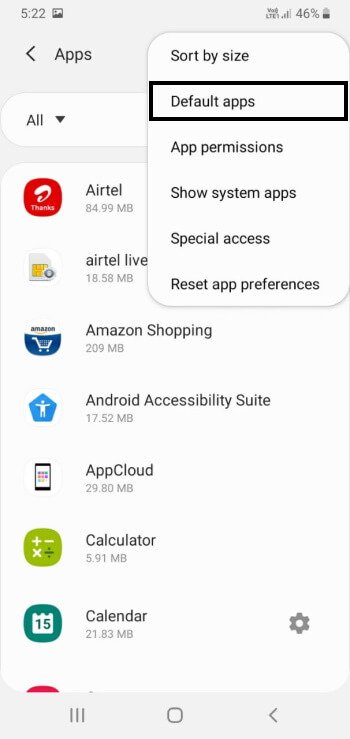The image displays a smartphone screen showing the "Apps" section of the device settings. It is 5:22 PM, and the phone's battery level is at 46%. At the top of the screen, a header reads "Apps" with a left-pointing arrow next to it. A pop-up menu is visible with the following options: "Sort by size," "Default apps," "App permissions," "Show system apps," "Special access," and "Reset app preferences." The "Default apps" option is highlighted with a black rectangle around it.

Below the pop-up menu, there is a dropdown labeled "All" and a search bar. The screen then lists several apps with their respective memory usage: Airtel (84.99 MB), Airtel Live (18.58 MB), Amazon Shopping (209 MB), Android Accessibility Suite (17.52 MB), App Cloud (29.80 MB), Calculator (5.91 MB), and Calendar (21.83 MB).

In the bottom right corner, there is a settings icon. At the very bottom of the screen, the device's navigation bar is visible, consisting of three colored icons: a line, a circle, and a back button, with colors red, blue, yellow, and green.